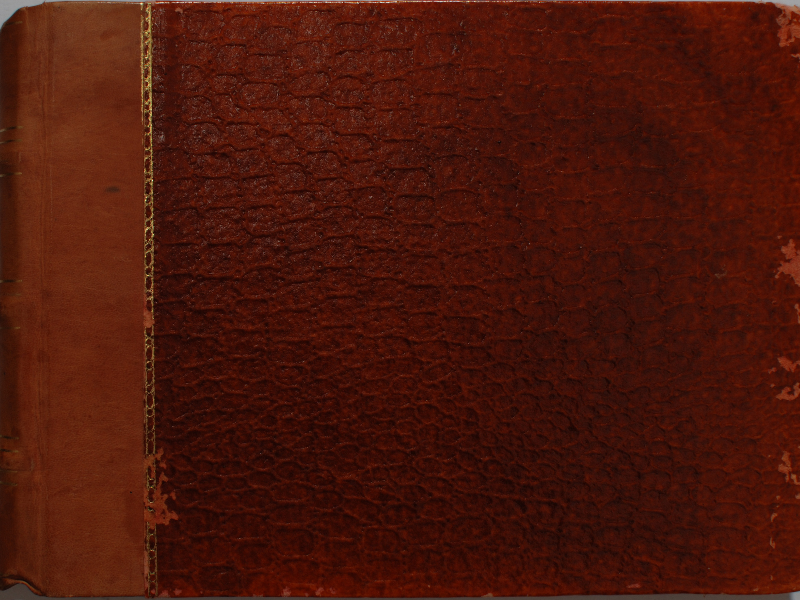This is a close-up photograph of a very old, bound book, captured in a macro style that emphasizes its textured leather surface. The book appears to be a reddish-brown or chestnut color, indicative of aged leather, and shows signs of flaking and distress, particularly around the edges and binding. On the left side of the image is the smooth binding, which features vertical gold lines running along its length. The top and bottom corners of the left side display patches of light gray, likely due to wear. Moving to the right, the leather transitions into a darker, crinkly texture with lines that vary in shades of dark red. This area resembles snake skin, though it may just be natural variations in cow or sheep leather enhanced by the close-up shot. The right-hand side of the cover has a few lighter reddish-brown patches similar to the far left, adding to the book's mottled, time-worn appearance. The very top corners reveal a white background, softly framed by the slightly rounded edges of the book.